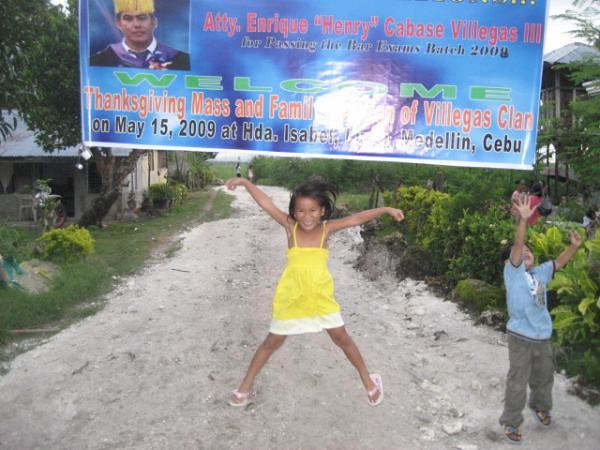In the photograph, a young Asian girl, dressed in a yellow dress with white trim at the bottom and pink flip-flop sandals, is captured mid-jump on a dirt road. She is the central figure in the image, energetically leaping into the air beneath a large blue banner that stretches across the road. The banner announces a Thanksgiving Mass and Family Reunion for the Villegas clan, featuring the name and picture of Enrique Henry Cabezas Villegas III. The event is dated May 15th, 2009, and located at Hda Isabel in Medellin, Cebu. To the girl's right, a young boy, possibly her brother, dressed in green pants and a blue shirt, also reaches up toward the banner, his hands extended high. The scene is set in a small neighborhood with houses and patches of grass on either side of the dirt road, suggesting a picturesque rural setting.